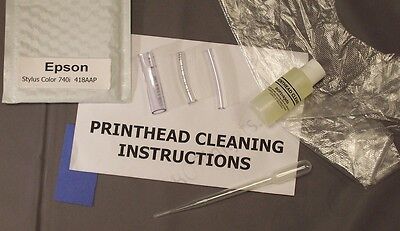The image depicts a brown table with several clear plastic tubes of varying lengths and thicknesses laid out. Prominently, there is a piece of paper with the title "Printhead Cleaning Instructions" and an Epson label indicating "Epson Stylus Color 740". Next to the paper is a small transparent bottle with a white lid containing a yellow liquid. Additionally, under the left side of the instructions paper, there's a rectangular blue piece of paper. The bottom part of the instructions highlights a dropper, and a piece of plastic is observed under the bottle in the upper right corner. The setup implies preparation for cleaning the print heads using the provided materials.